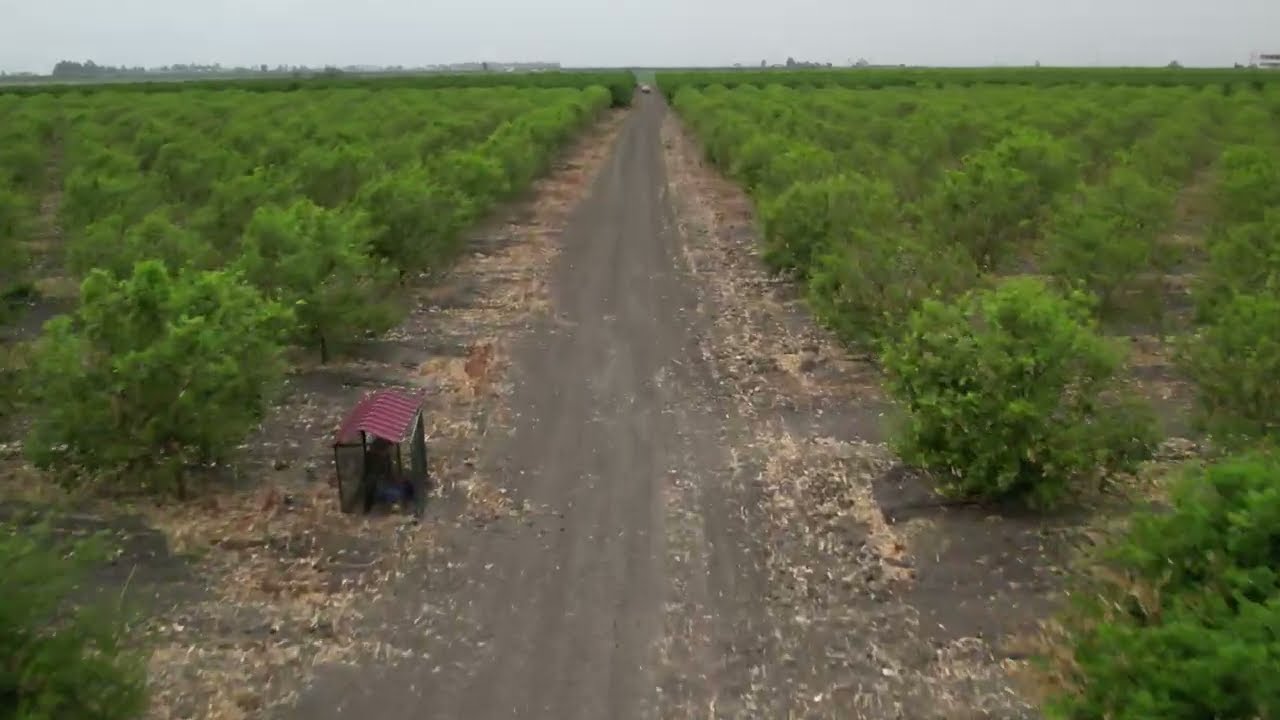This rectangular photograph, taken from an elevated, angled perspective, showcases a lengthy dirt and gravel road extending from the bottom to near the top of the image. The road is flanked by rows of bright green, round trees, suggesting a meticulously planted orchard. Approximately in the middle of the image, positioned on the left side of the road, is a small structure resembling a bus stop, featuring a dark-colored, possibly fine-caged or glass enclosure and a red, corrugated metal roof. The sides of the structure are open, adding to the ambiguity of its purpose. Along the edges of the road, there's a mixture of tan-colored material, possibly rocks or dried plants, blending with the gray dirt. In the far distance, a vehicle can be seen driving down the center of the road, too small and far to discern clearly. Beyond the orchard, the background reveals faint outlines of distant buildings or maybe mountains under a strip of light gray sky, completing this serene yet detailed landscape.